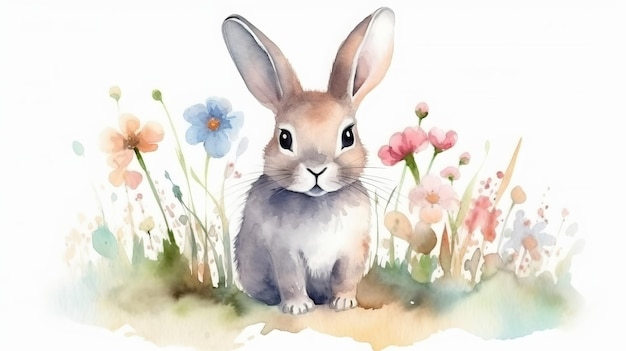This artwork is a detailed watercolor painting of a youthful bunny with long ears and a puffy face. Rendered in shades of light brown with a white chest and white patches surrounding its large, expressive black eyes, the bunny is portrayed with its two front paws and whiskers clearly visible. The bunny's eyes are wide open, featuring a glossy reflection, and it has a delicate nose and mouth. The scene is set in a vibrant garden where the bunny is surrounded by a variety of flowers—blue, orange, different shades of pink, and some green and yellow blooms. The flowers are tall and thin, encircling the bunny, which sits at the center of this colorful patch. The overall demeanor of the bunny is neutral, facing directly forward without any distinct expression, imparting a sense of calm and innocence. The absence of other elements like people, shadows, or indications of time of day, along with the cartoonish and slightly whimsical style of the piece, makes it ideal for display in a living area or a bathroom.